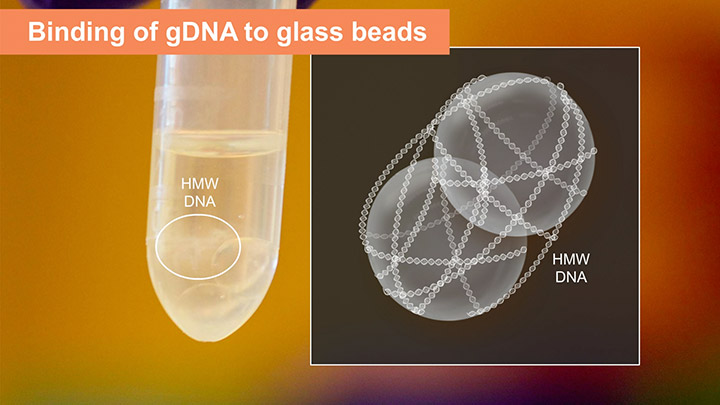This detailed poster, potentially sourced from a biology textbook or a resource focused on heredity and DNA studies, exhibits a chemical process. Dominated by a distinctive color gradient background transitioning from yellow to dark red, the image is split into two main sections.

On the left, a photograph captures the bottom part of a test tube, which contains approximately three-quarters of an inch of fluid and several glass beads settled at the bottom. Above this image lies an orange bar labeled "Binding of gDNA to Glass Beads," suggesting the procedure depicted.

To the right, a dark gray square showcases an illustration labeled "HMW DNA." This section features two glass beads encapsulated by numerous DNA chains in various orientations, symbolizing the binding interaction between the gDNA and the glass beads.

The notable visual elements include the liquid and bead-filled test tube on the left and the detailed representation of DNA-bead interaction on the right, both set against a striking yellow-to-red gradient and a dark gray square backdrop, respectively.